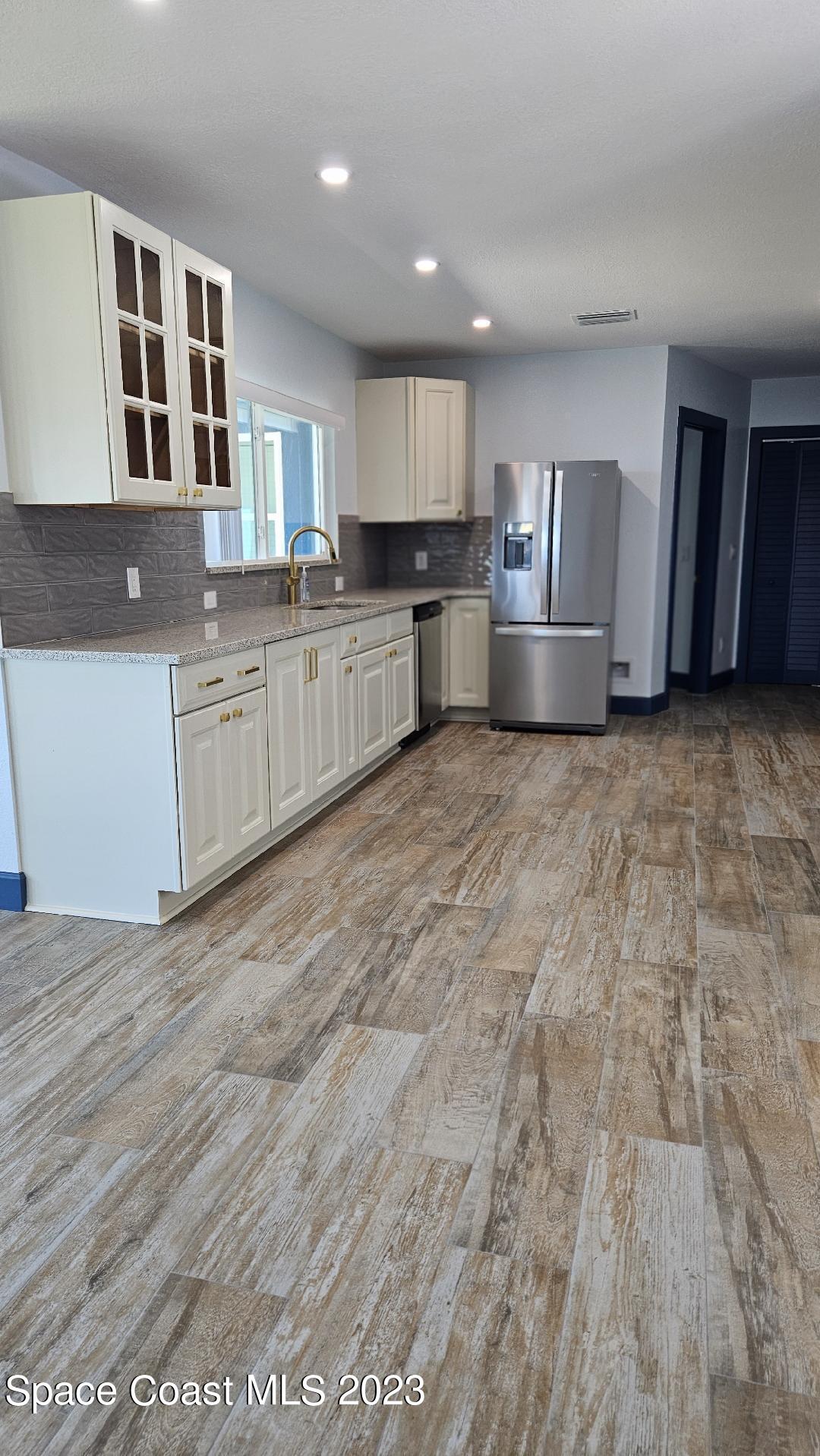This meticulously staged commercial photograph showcases a modern kitchen, likely part of a for-sale or for-rent property, as indicated by the "Space Coast MLS 2023" text in the bottom left corner. The kitchen features sleek white cabinetry on both the upper and lower levels, accentuated by elegant gold hardware. A luxurious stone countertop extends diagonally from the left side towards the center of the frame, housing a centrally placed sink with a striking gold faucet. Above the sink, a window offers natural light, complemented by additional cabinetry. To the right of the sink, a silver refrigerator stands prominently against the wall, juxtaposed beside an air return duct—a peculiar placement in the otherwise harmonious design. The backsplash consists of textured, dark gray subway tiles, adding depth and contrast to the space. The floors appear to be vinyl or wood-like tile with a concrete finish, enhancing the modern aesthetic. The ceiling features three spotlights, casting a warm glow throughout the room. Two doors are visible in the background, one of which may lead to a pantry, garage, or outside area, adding functional versatility to the stylish kitchen space.